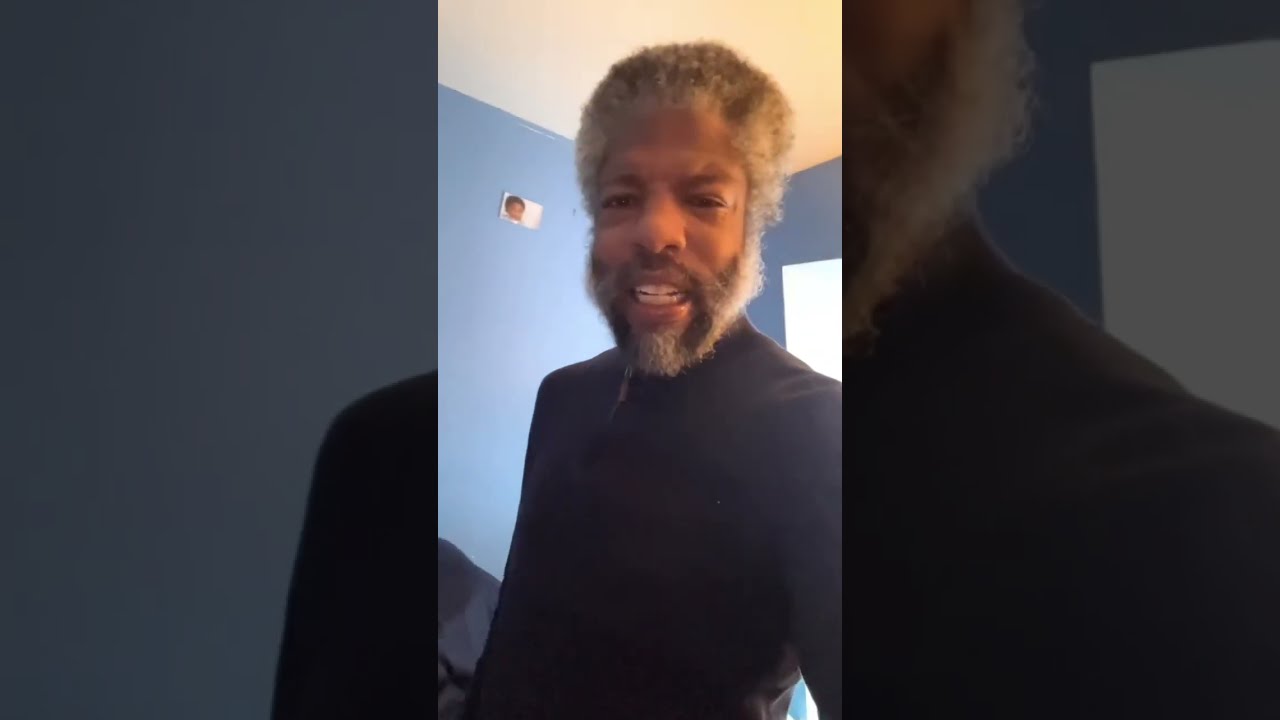In this multifaceted photo, a dark-skinned male is slightly smiling or possibly speaking as he takes a selfie, extending his left arm into the foreground. His distinguished salt-and-pepper hair forms a fluffy texture atop his head and complements his medium-length, patchy gray beard and mustache. He's dressed in a black long-sleeve shirt or a blue turtleneck sweater that zips at the front, standing in a room with calm blue walls and a white ceiling. Background details include a small photo of a young child affixed to the blue wall, adding a subtle personal touch. The unique composition features three panels: the central image of the man from chest up with his stretched arm, and the outer panels zooming in on specific portions of the main picture. The blue of the wall is distinctly lighter than his shirt, framing the serene yet intriguing scene captured in this moment.